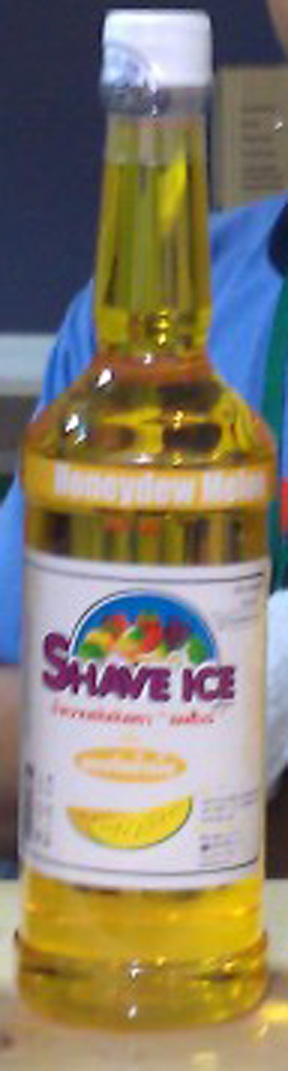A clear bottle filled with a yellow liquid prominently features a label saying "Shave Ice." The label's design includes an array of fruits, such as grapes, an apple, a banana, and what appears to be a yellow lime near the bottom, likely indicating the flavor of the contents. The label itself has a clean, white background. The bottle is set on a white table, suggesting a clean and minimalistic setting, possibly within a bar or similar establishment. Behind the bottle, a person in a blue shirt is partially visible, seated against a blue wall, reinforcing the notion of a public venue where such a product might be served.